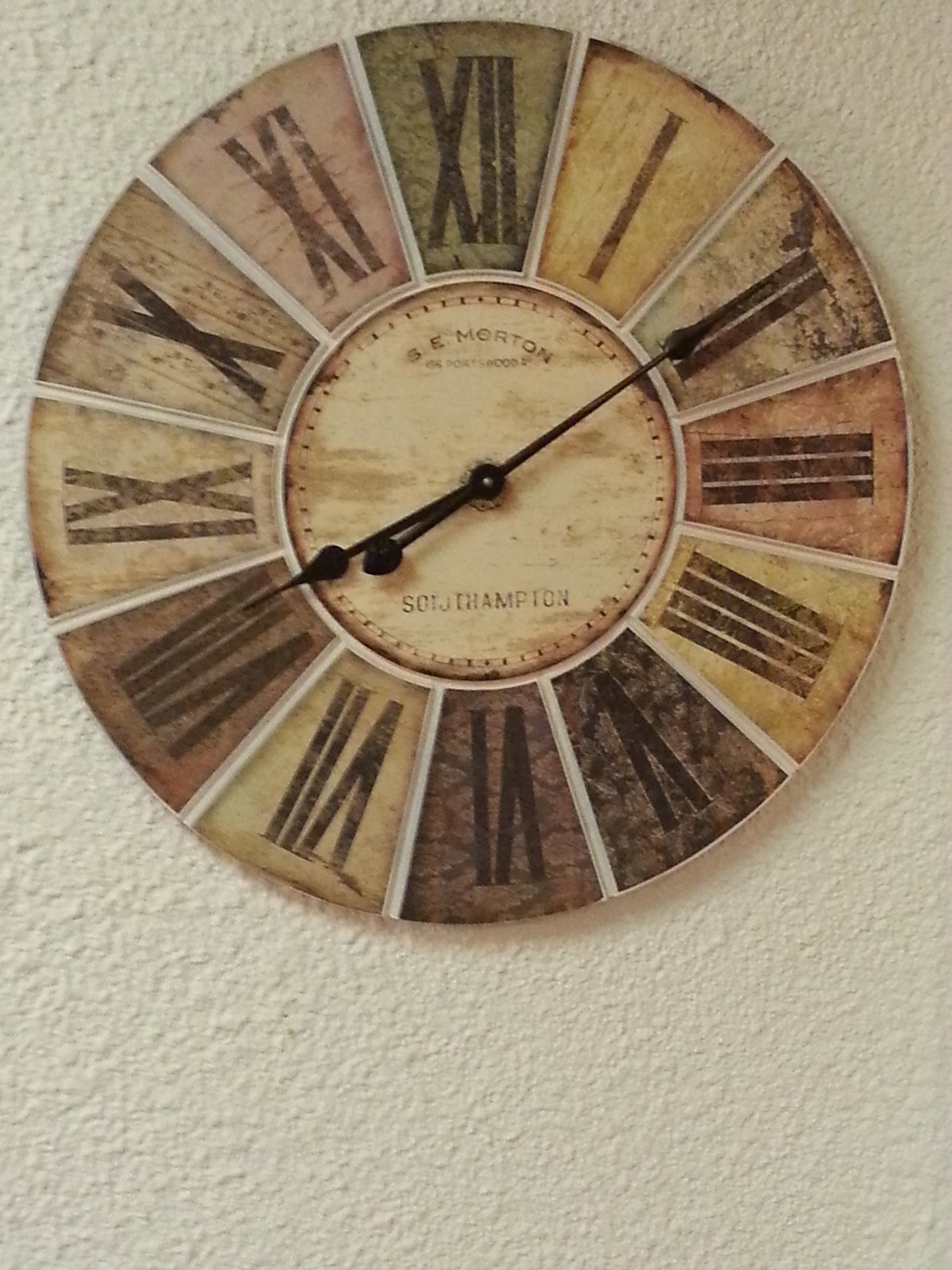An antique-style clock, featuring a distressed, multi-colored finish in hues ranging from off-white to yellow, dark brown, hinting of red, and subtle green, is mounted on a rough-textured, off-white wall. The clock is adorned with elegant Roman numerals and has three hands: hour, minute, and second. The top of the clock is inscribed with "S.E. Morton" accompanied by smaller, less legible text beneath it. "Southampton" is prominently displayed at the bottom, adding to its vintage charm.